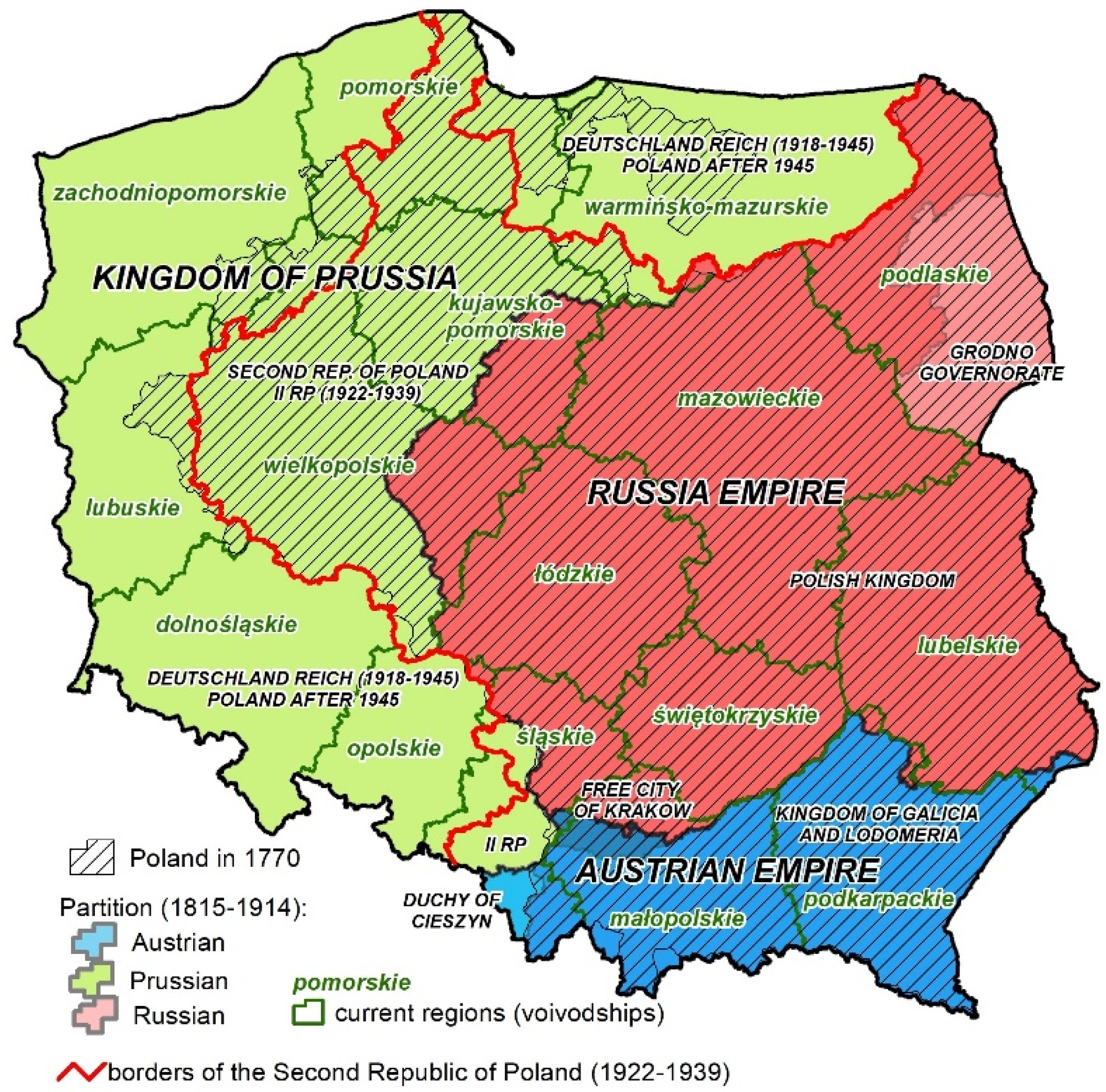This is an image of a political map highlighting the territorial divisions of Poland in 1770. The map distinctly outlines three major empires using different colors: the Kingdom of Prussia in green, the Russian Empire in red, and the Austrian Empire in blue. Each empire's name is labeled within its respective color-coded area. Notable regions include the Kingdom of Galicia and Lodomera within the Austrian Empire, as well as a tiny light blue section marked as the Duchy of Cieszyn. The map also features a legend at the lower left corner, detailing the meaning of each label and color. A prominent red line indicates the borders of the Second Republic of Poland from 1922 to 1939. The map focuses solely on political boundaries, without depicting any geographical features like mountains or rivers.